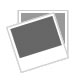The image captures a detailed view of a textile artwork, possibly a felt pennant or rug, spotlighting a caricature of a Los Angeles Dodgers pitcher in mid-windup. The pitcher, adorned in a distinctive blue cap with "LA" and a white jersey emblazoned with "NOMO 16" in blue, stands in an exaggerated pose with his left leg raised and body twisted, ready to throw the ball from his black mitt. The character sports white pants, a white and black belt, and white and blue cleats, all meticulously illustrated. Below the player's name and number, two red Japanese characters are featured, adding an international flair. The artwork, signed by the artist Mudge, prominently displays a dynamic background; the top half rendered in white resembling a whirlwind effect, transitions into a gray middle ground and culminates in a darker bottom section. The left edge of the textile is marked by a black border, and additional text reads "Wincraft, made in USA." The entire scene is set upon a dark brown hardwood floor, emphasizing the wood grain visible above and below the pennant.